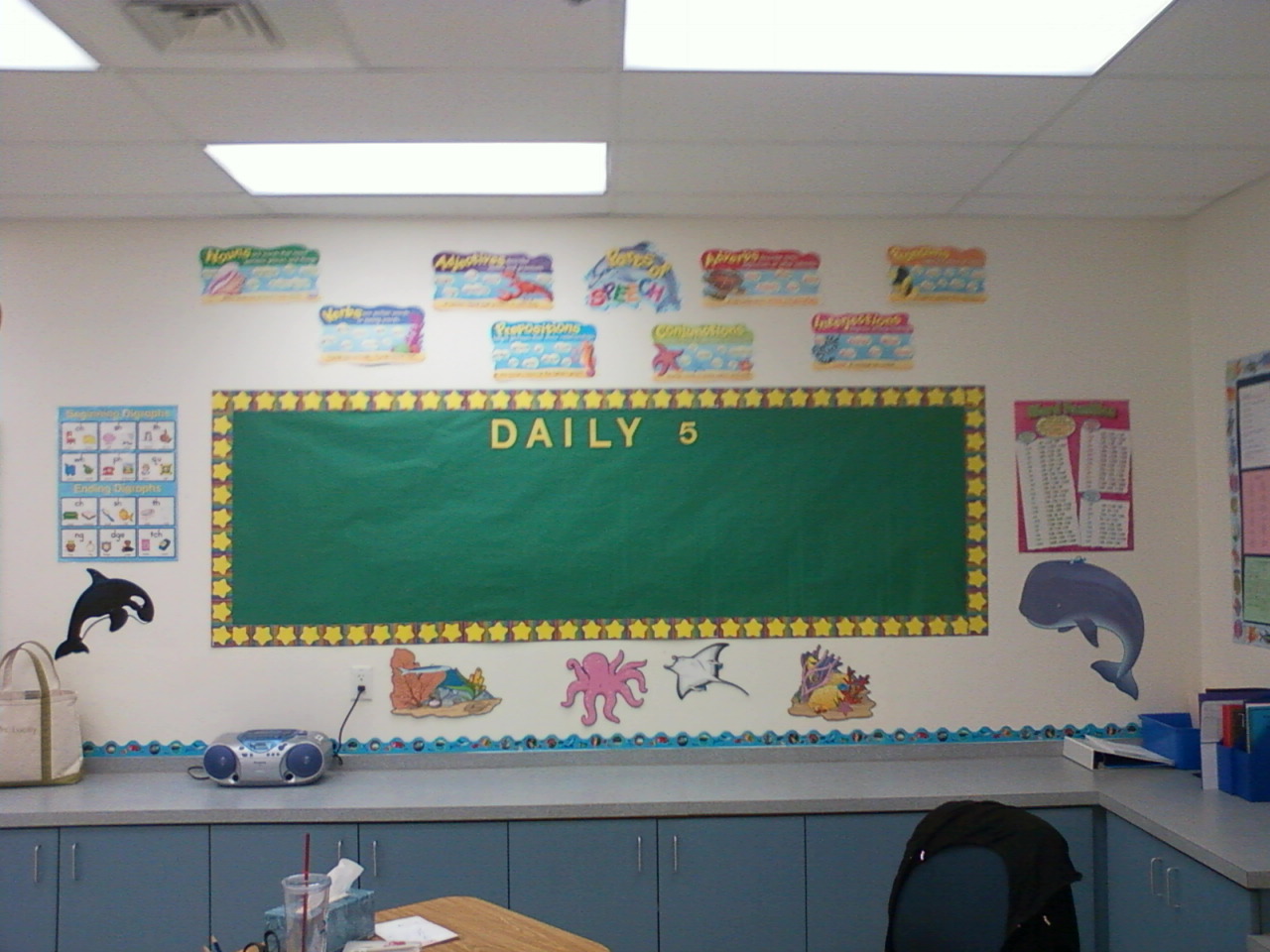This color photograph captures a detailed corner of an elementary school classroom, immediately drawing the eye to a large green butcher paper rectangle tacked to a white wall. This green area, bordered by bright yellow stars, prominently displays the words "daily 5" in bold yellow letters. Surrounding this central feature are various stencils and decals of sea creatures, including an orca (killer whale), an octopus, a manta ray, and a blue whale. Additional smaller, colorful sketches of various scenes with words decorate the wall above. Below this vibrant display, a large gray countertop extends along the wall, housing various blue cabinets with silver handles. Atop the countertop, a portable stereo radio is plugged into an outlet, emphasizing the functional aspect of this lively, educational space. This scene vividly illustrates the creative and organized environment typical of an elementary school classroom.